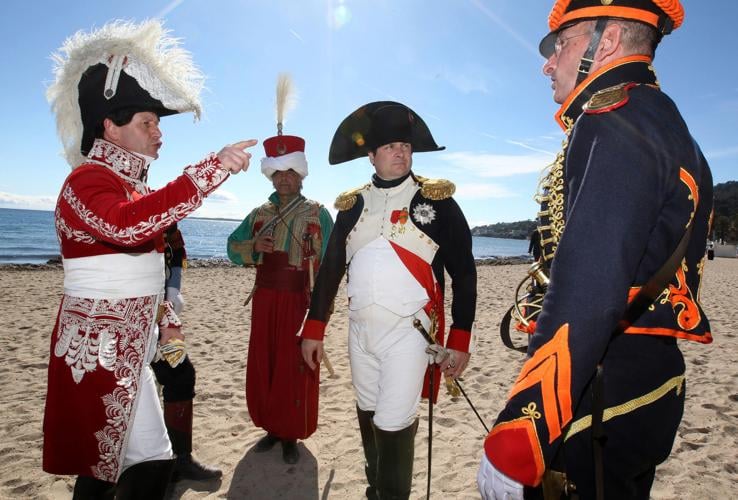The image depicts four men standing on a sandy beach with the ocean in the background under a bright blue sky with a few wispy clouds and rays of sunlight. They appear to be dressed in various historical or ceremonial military uniforms. The man on the far left wears a red coat with white embellishments, white pants, and a black hat adorned with a long plume of white feathers. He seems to be pointing and possibly yelling at another man. The second man, who appears to resemble Napoleon, sports a uniform that looks distinctly French, including a Napoleon-style hat, and carries a sword. The third man is dressed in red pants and a green and yellow long-sleeved shirt, topped with a red hat featuring a large feather. The fourth man, closer to the center, dons a navy blue and orange uniform with gold accents, complete with a matching hat and a sword at his side. The scene conveys a sense of dramatic tension and historic or martial importance.